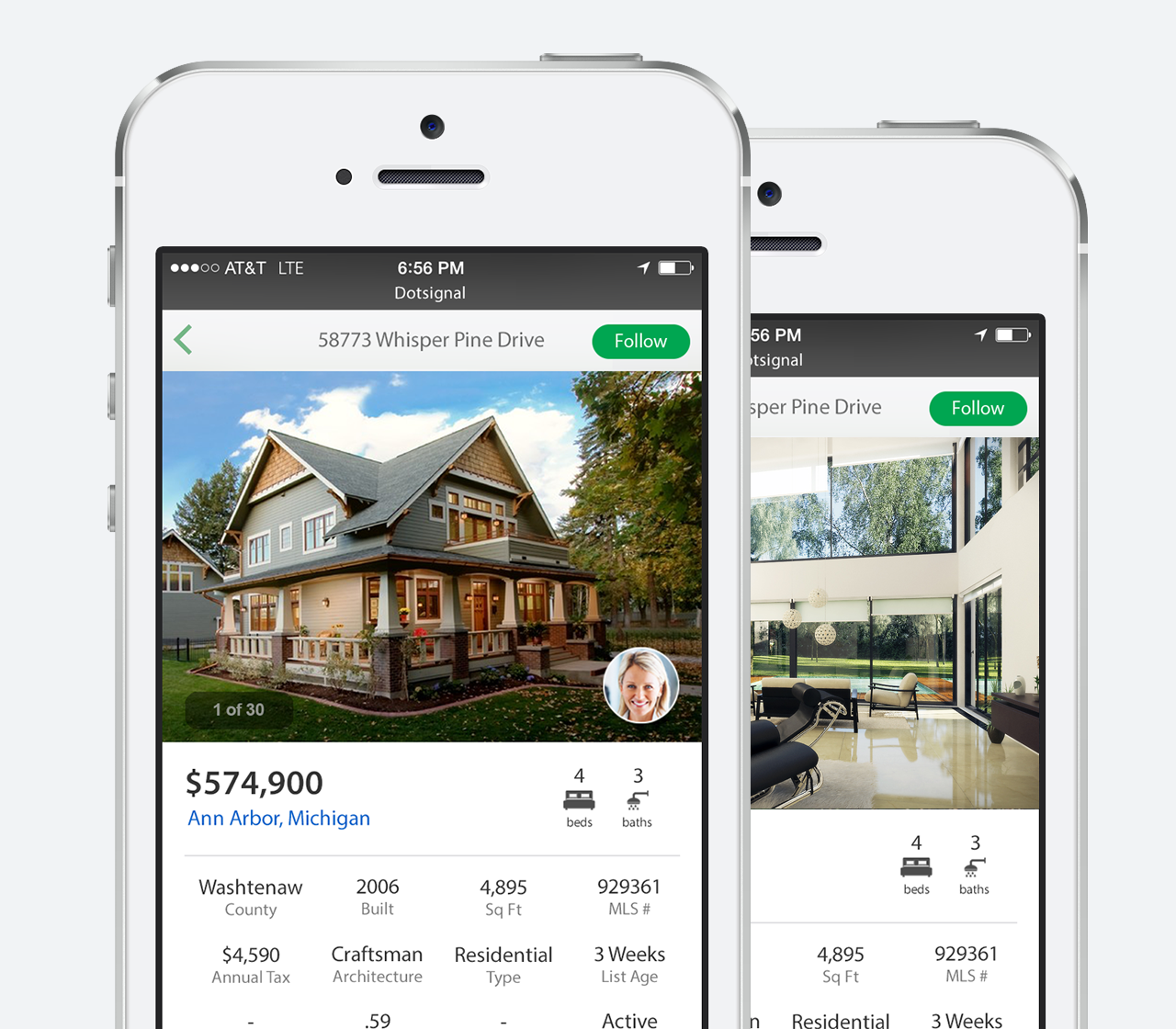The image depicts two iPhones displaying listing details for a house on Whisper Pine Drive, Ann Arbor, Michigan, with the address 58773. Both phones show the time as 6:56 PM, and they are connected to AT&T service. The left phone displays an exterior image of a two-story Craftsman-style house with a wraparound porch and an interesting roofline. The house is listed for $574,900 and has been on the market for three weeks. The right phone showcases an interior shot of the same house.

This property is 4,895 square feet, featuring four bedrooms and three bathrooms. Built in 2006, it is located in Washtenaw County and has an annual property tax of $4,509. The MLS number for this listing is visible, ensuring ease of reference for prospective buyers. A professionally photographed image of a woman, presumably the real estate agent, is also shown in front of the house. The devices capture the essence of someone engaged in high-end house shopping.